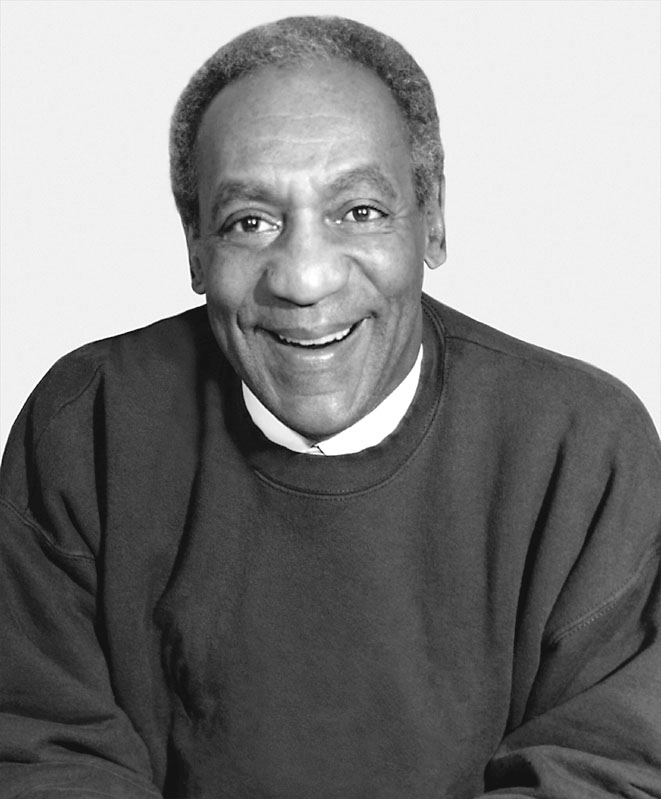This is a detailed, black-and-white headshot of a slightly older Bill Cosby, showcasing his signature smile. Cosby is dressed in a dark, unpatterned sweatshirt that shows subtle wrinkles, indicating its clean texture, and underneath, he wears a white collared shirt. His hair, a thick and curly mixture of gray and black, recedes slightly towards the back. In the image, he appears to be seated with his arms possibly resting in front of him, adding a relaxed demeanor to his pose. The background is plain and light-colored, possibly white, enhancing the focus on Cosby. There's a light source illuminating the center of his face, giving it a brighter appearance compared to the rest of the image, which further accentuates his smile.